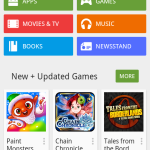This cropped and slightly blurry image depicts a section of the Google Play Store, showcasing its navigation categories and new game offerings. The screen highlights six main categories, each represented by vibrant color-coded buttons: green for Apps and Games, orange for Music, red for Movies and TV, and blue for both Books and Newsstand. Below these categories, the "New and Updated Games" section features a selection of app covers and titles. Among them are "Tales from the Borderlands," which is depicted with a text-heavy cover, "Paint Monsters," illustrated with a cheerful, childlike red monster character, and "Chain Chronicle," which features an androgynous teenage character gazing towards the viewer. The image cuts off just around a 'More' button, hinting at additional content beyond the visible portion.